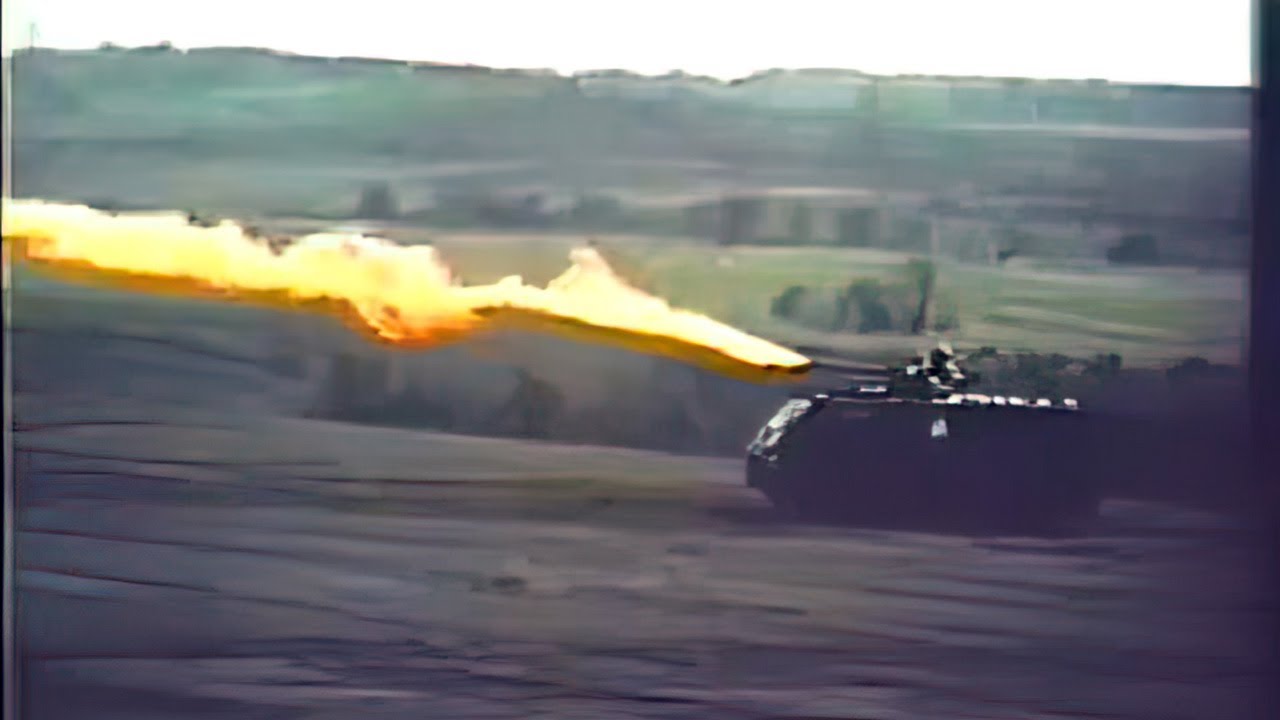The image depicts a blurry outdoor scene centered on a tank situated in a field with a dark, possibly dirt-covered ground. Despite its indistinct nature, the tank is noticeable on the right side of the image, with its turret firing a vivid burst of bright yellow and white flames from the barrel. The tank is partially shrouded in shadow, making it challenging to discern if it's a real photograph or a digital rendering. There appear to be faint silhouettes of trees and greenery in the distant background, adding to the smoky and obscure atmosphere of the scene. Additionally, a person may be seen standing on or near the tank, although their features are not clear. The blurry landscape in the background features low hills and a white sky, contributing to the overall indistinct and dim setting. A black strip runs down the right side of the image, suggesting it might be a frame from a film or a cropped screen.